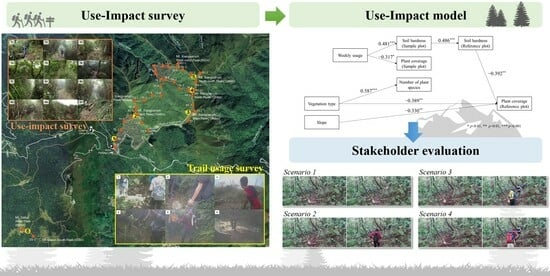This detailed photographic image, likely taken from a presentation, showcases a series with two main components: the "Use Impact Survey" on the left and the "Use Impact Model" on the right. The left side features a green valley-like topographical map with yellow markings and labels, illustrating people with backpacks and canes walking along a trail. Above this map is an insert of twelve small photos in a grid, marked "Use Impact Survey," with diverse visuals, including individuals wearing red and white backpacks and various landscapes. In the bottom right corner of this section is another inset titled "Trail Usage Survey," displaying six images of people, hands, trees, shrubs, and bushes.

On the right side, the "Use Impact Model" includes a detailed flowchart consisting of eight interconnected boxes and arrows, and a graphic of mountains in the middle section. Each box contains text and possibly numbers, but these details are too small and blurred to read clearly. Among these interconnected elements, a blue arrow points downwards to a box labeled "Stakeholder Evaluation," emphasizing the involvement of various participants in the survey model. Below, four scenarios are presented in two rows, each containing four images primarily of trees and one recurring individual with a red backpack, reflecting different observational results. The combined imagery and intricate design suggest thorough research and complex data visualization, underscoring its presentation-like quality.